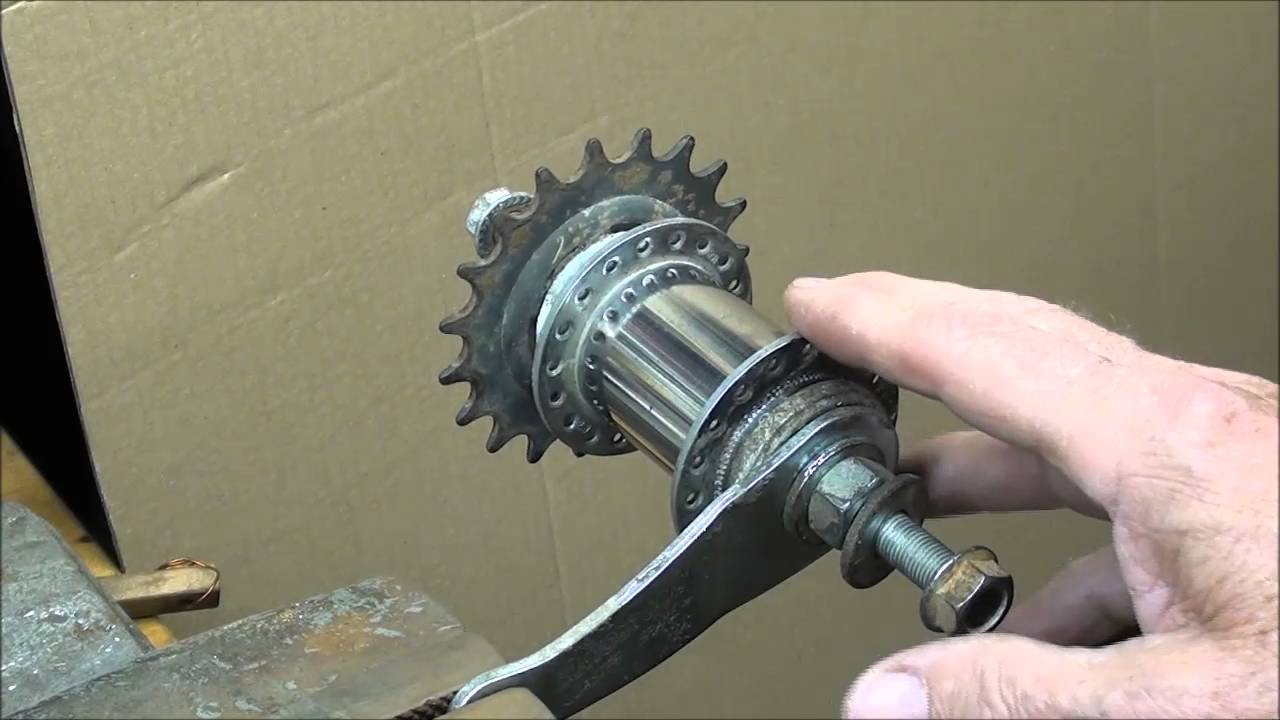In the photograph, an elderly hand with visible hair is seen grasping a mechanical component. The component, resembling a bicycle's rear wheel cassette, features a series of three metal gears with circular teeth, suggesting it might be a spoke or bike gear. The cylindrical part of the contraption is held together by a nut and bolt, and it is mounted on a vise with a rust-colored finish. The hand holds the cylinder with the thumb and fingers touching the gears. The background reveals a workbench made of tan-colored wood against a brick-tan or cardboard wall, adding to the vintage workshop atmosphere. An adjacent brass piece with attached wires hints at other tools or equipment in the setting. The detailed image captures the essence of hands-on mechanical work, focusing on the intricate components of a bicycle's gear system within a rustic workspace.